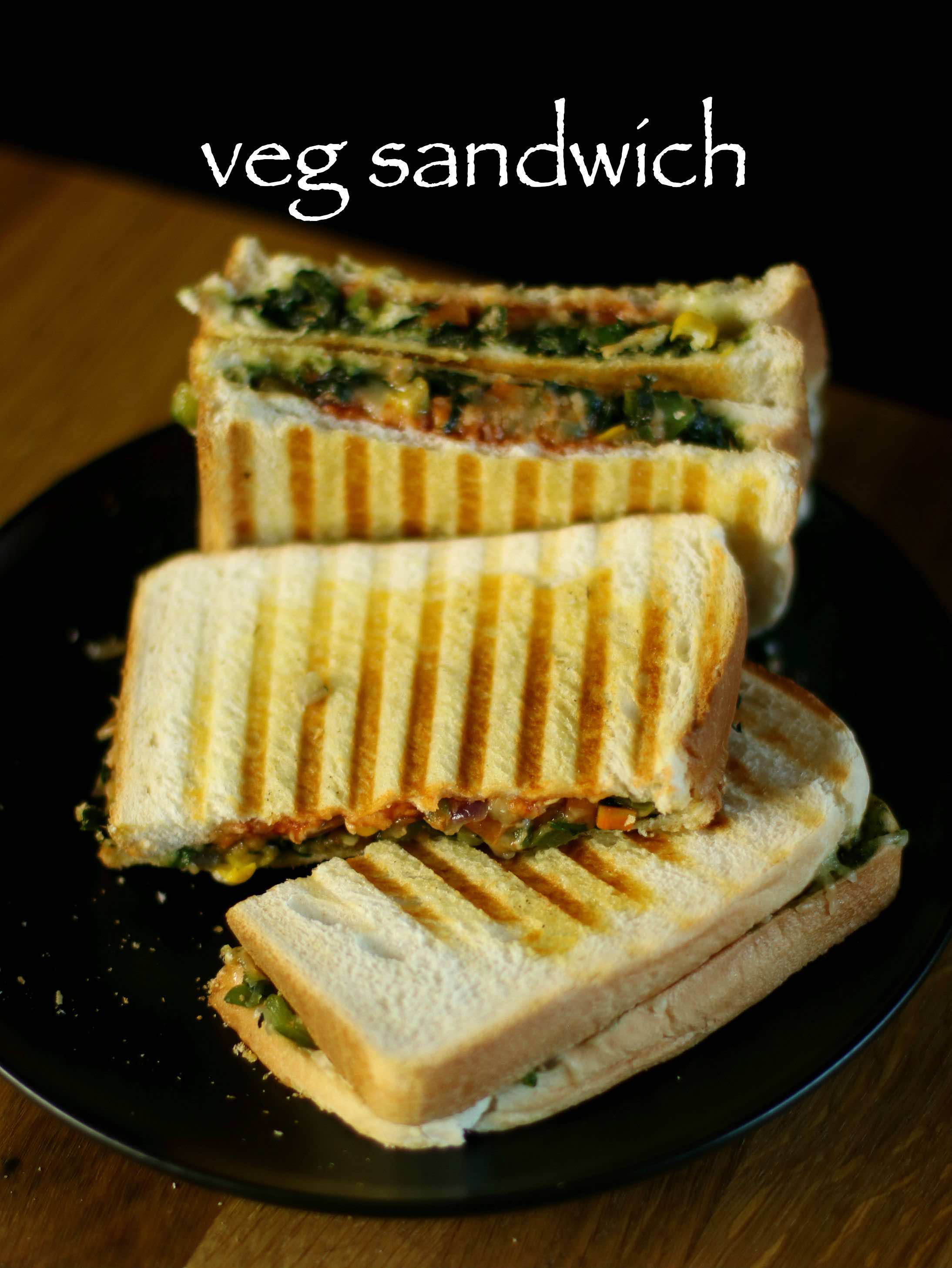In this vertical image, we observe a detailed close-up of a grilled vegetable sandwich, labeled "VEG sandwich" in white at the top of the frame against a black background. The sandwich is presented on a round black plate situated on a medium-brown wooden table, which appears at the bottom edge of the image. The two sandwiches are cut in half, with varied positioning to highlight their contents. The back two halves are stacked upright at roughly a 45-degree angle, exposing the vibrant fillings of spinach, tomatoes, artichokes, and possibly other vegetables in shades of green, red, brown, orange, and yellow. The front half is laid flat, while another piece leans against it and the upright halves, creating a layered, dynamic display. The bread is white with noticeable grilled, yellowish-brown lines, likely from a panini press, adding a rustic, appetizing texture to the overall presentation.